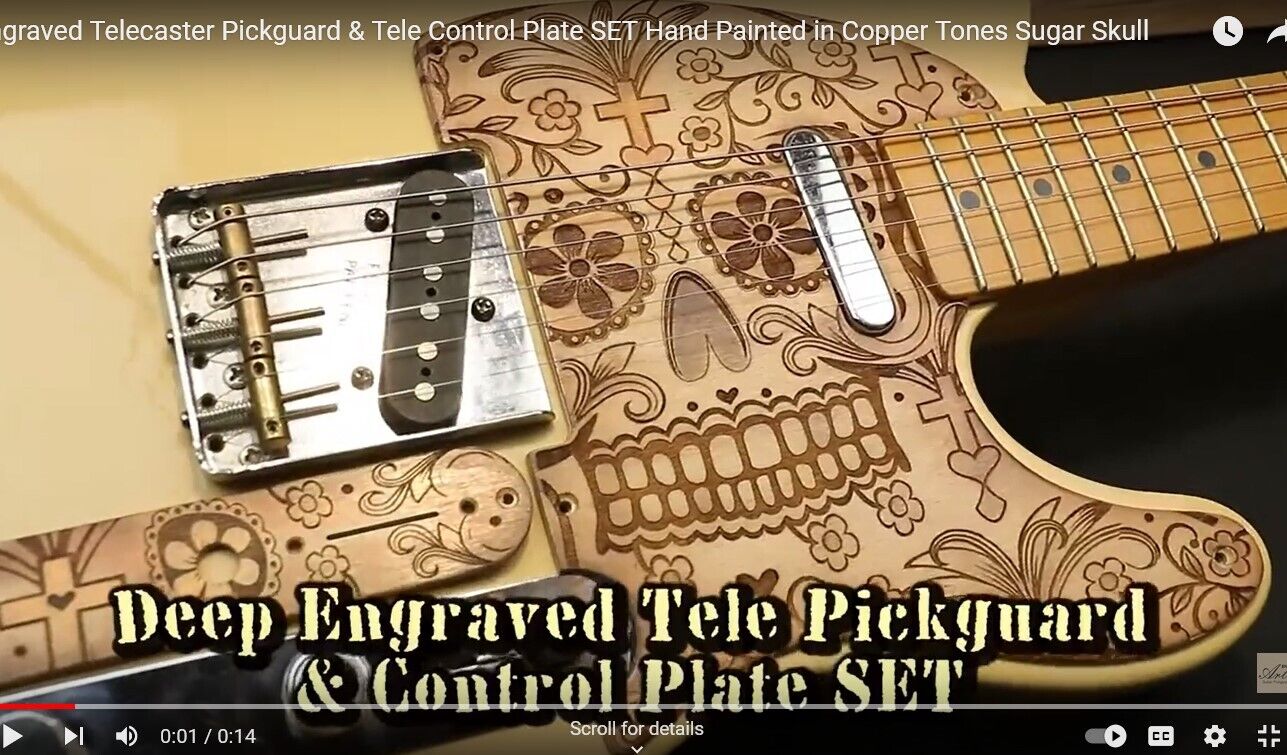The YouTube thumbnail image depicts an ornately designed Telecaster guitar engraved in light tan and light brown wood textures. This intricate design features a prominent sugar skull motif, evocative of Dia de los Muertos celebrations. The skull is adorned with detailed floral and cross engravings, specifically with flowers in the eye sockets, a cross above the nose bridge, and a heart beneath the cross. The design continues with teardrop shapes descending from the nose area, and intricate patterns including diamonds, additional hearts, and floral elements are scattered around the skull. The engraving itself is unpainted, allowing the darker wood tones to accentuate the design intricacies. The image background is black, highlighting the guitar's details. The screen also contains typical YouTube interface elements like play, skip buttons, volume control, and captions. Text overlays in white and yellowish lettering read: "Graved Telecaster Pickguard and Tele Control Plate Set Hand Painted in Copper Tones Sugar Skull" and "Deep Engraved Tele Pickguard and Control Plate Set."